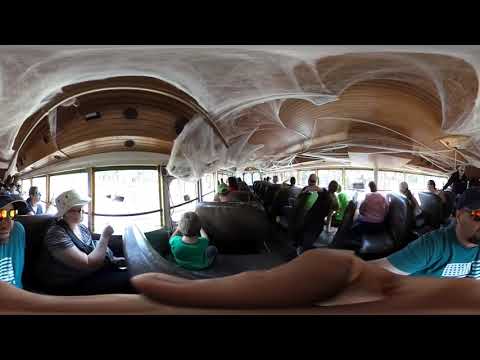This panoramic, 360-degree image captures the interior of a sightseeing tram with a fully wooden interior ceiling accented by white mesh material. The photographer, visible in the shot, sports sunglasses, a black hat, a neat French beard, and a light blue t-shirt featuring a white American flag design. He holds the camera with his right hand, and his fingers are partially visible at the bottom of the frame.

Next to him, a woman wearing a short-sleeved blouse and a white hat with glasses seems engrossed in the scenery outside, her attention mirrored by a young boy in a green shirt sitting in front of her, also captivated by the outside view. Along the aisle, numerous other passengers are seated, most of whom are intently gazing out the bright windows, indicating that the tram is likely on a scenic route. 

The atmosphere inside the tram is bustling with curiosity and excitement as people are leaning and pointing to catch a glimpse of the sights outside. Despite the brightness outside making it difficult to discern what everyone is looking at, the shared sense of interest among passengers underscores the purpose of the vehicle as a shuttle for sightseers, making leisurely rounds and offering picturesque views along the way.